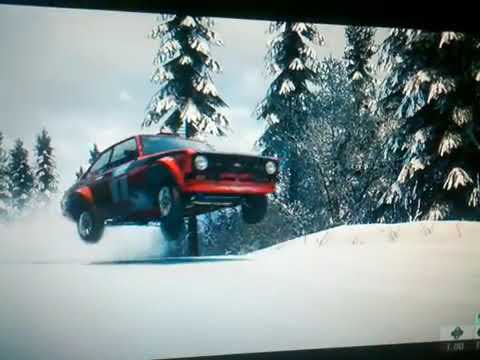The image captures a snow-covered landscape featuring a red and black compact car, possibly a rally car, mid-jump with all four wheels off the ground. The car kicks up snow as it leaps through the air, suggesting high-speed action. In the background, a mix of snow-dusted pine trees stretches beneath a mostly cloudy sky. The terrain appears to be a snowy off-road course, with some grass shoots peeking through the snow. The car, which has a silver racing stripe down its passenger door and a flat front grille with round headlights, looks like a vintage model from the 1980s. The image itself seems to be a photograph of a computer screen showing a scene from a video game, hinted by the uneven black borders and the slightly unrealistic appearance of the trees. In the bottom right corner of the screen, there is a green logo and some text, reinforcing the idea that the scene is from a digital game.